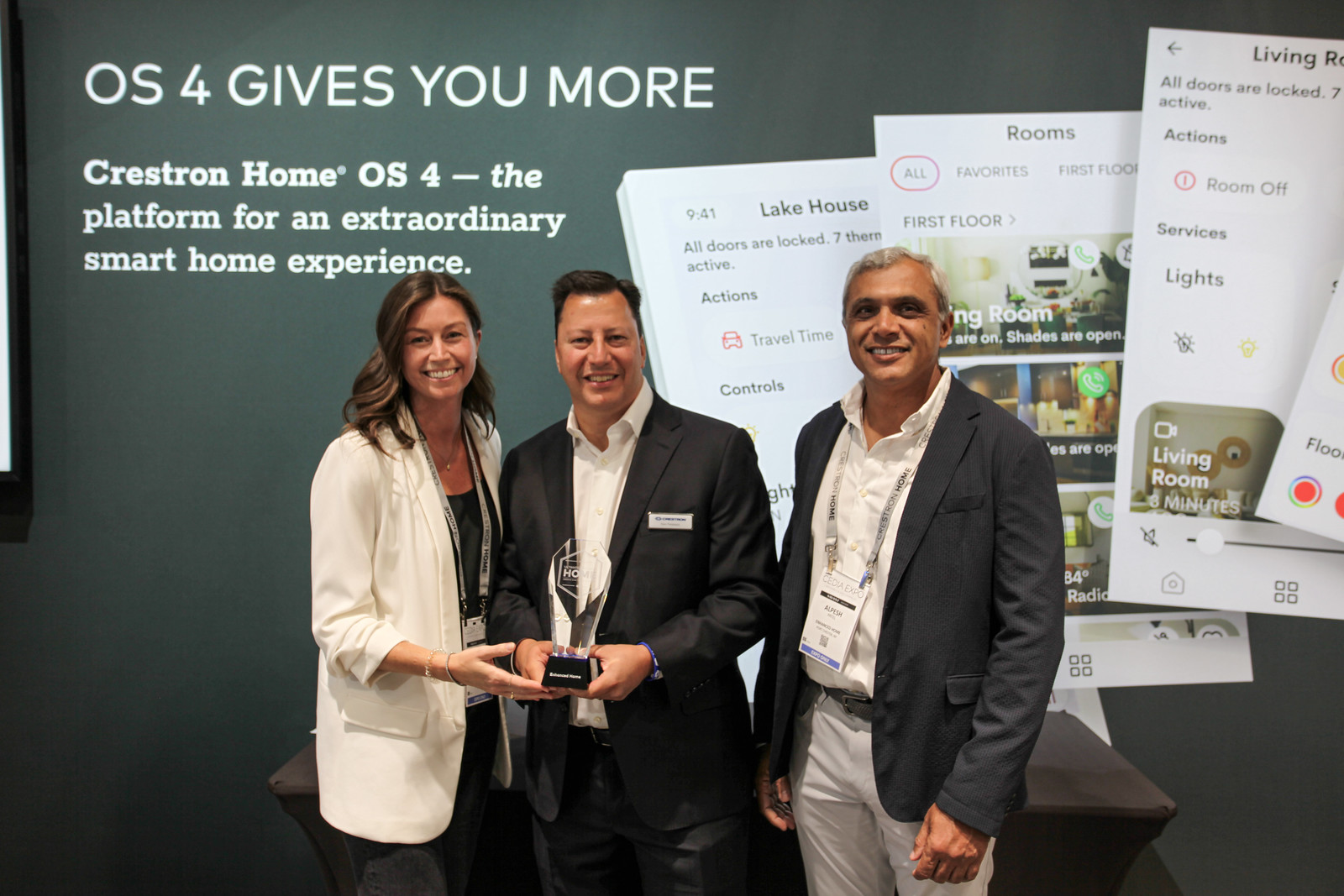The image is an indoor advertisement for Crestron Home OS4, showcasing its tagline, "OS4 gives you more: the platform for an extraordinary smart home experience." In the center of the rectangular photograph, which is wider than it is tall, stand three individuals from mid-thigh up. To the left, a young woman with light tan skin and curled brown hair, wearing a long-sleeve white dress jacket over a dark shirt, is smiling as she supports a trophy. Next to her is a man of similar height and complexion, dressed in a dark gray suit jacket with a white button-up shirt, holding the black and glass trophy. To his right stands an older gentleman with brown skin and white hair, clad in a lighter gray dress jacket, white button-up shirt, and white pants. All three are smiling at the camera, celebrating the recognition Crestron Home OS4 has received. Behind them, a grayish-blue wall displays the advertisement's slogan in white print and includes several images of home app pages, illustrating features like "lake house rooms" and "living rooms."